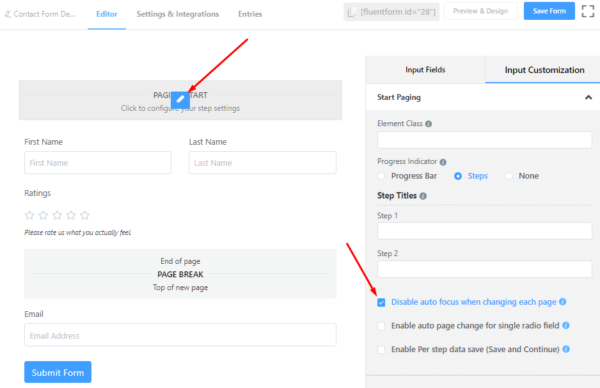In the image, the top left corner displays the text "Contact Form Developer" in black, followed by "Editor" which is highlighted in blue. Options for "Settings" and "Integrations" are also present. On the top right, two buttons labeled "Preview" and "Design" are visible; the "Save Form" button is blue and prominently placed.

The center of the image features a pen icon on the right side and a blue pen button on the left side, indicated by a red arrow. Form fields for "First Name" and "Last Name" are present, along with a section for ratings that says, "Please rate us on what you actually feel."

At the bottom of the page, there is space for an email address and a blue "Submit Form" button on the bottom left. The right side of the image includes a section for input customization options, with "Input Customization" highlighted in blue and underlined. Below this, it says "Start Paging" with an element class input field. 

There is also a progress indicator showing options like "Progress Bar" and "Steps," with "Steps" selected. Step titles "Step One" and "Step Two" have empty spaces for input. Three checkboxes are found on the bottom right, with the first one highlighted in blue and indicated by a red arrow. The options for the checkboxes are: "Disable auto-focus when changing each page" (checked), "Enable auto-page change for single radio field," and "Enable per step data save & save and continue."